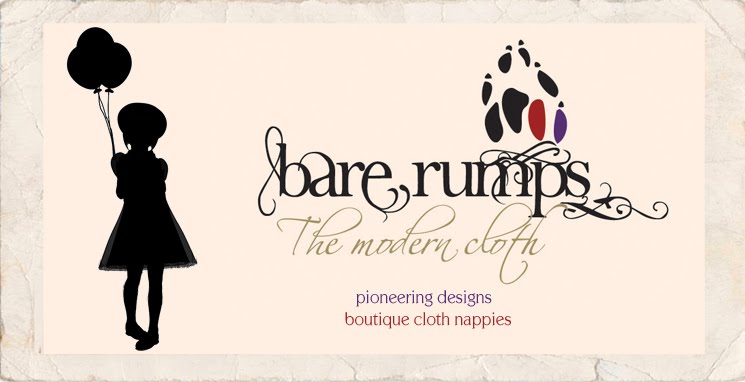This image is an advertisement featuring a rectangle layout with a weathered, lighter tan border framing a peach-colored inner rectangle. On the left side of the advertisement, there's a digital shadow silhouette of a little girl dressed in a hat and dress, holding three balloon strings, all depicted in black. Above her, the border showcases various footprints, mostly in black with some in red and a purple shape interspersed. 

To the right of the girl, the text is arranged in elegant black lettering with ornate lines and swirls, reading "Bare Rumps." Directly beneath this, in light gray, it says "The Modern Cloth." Further down, in purple lettering, it reads "Pioneering Designs," followed by "Boutique Cloth Nappies" in pink letters. The design overall combines intricate fonts and whimsical imagery to create an attractive and artistic advertisement.